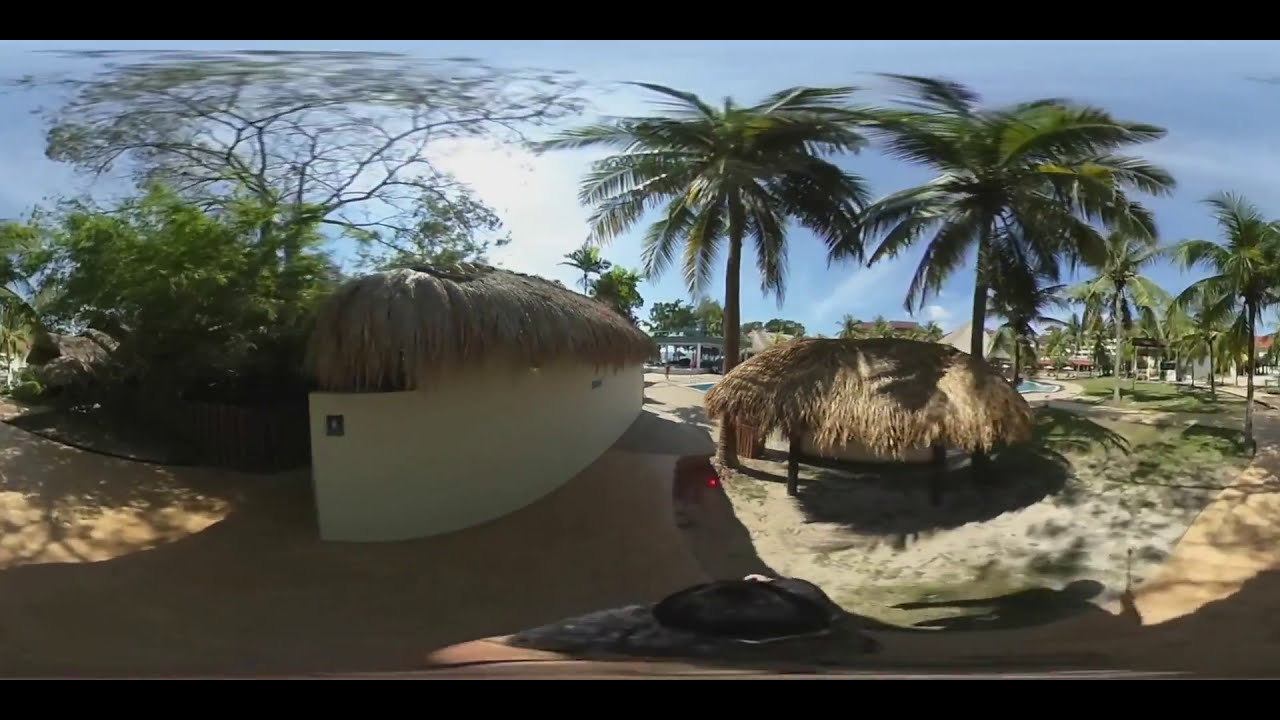This photograph captures a vibrant, summery beach scene dominated by lush palm trees and hut structures with straw roofs. At the center, a small gray wooden hut with a straw roof invites relaxation, standing adjacent to a similar structure that appears to be a restroom, identifiable by its curved white wall and a sign indicating its purpose. The pathway leading to the restroom is paved with beige tiles, blending seamlessly into the surroundings. The background features a blue sky, mostly clear with a few clouds, suggesting a bright, sunny day. There's a faint white patch in the sky, likely the sun, and patches of blue on the ground hinting at the possible presence of a pool. Despite the apparent tranquility of the scene, hinting at a public setting, there's minimal human activity visible, with the faint sighting of a person near the restroom and a couple of indistinct figures in the far background. This inviting vista is complemented by rows of palm trees that line both sides of the walkway, reinforcing the tropical ambiance of the locale.